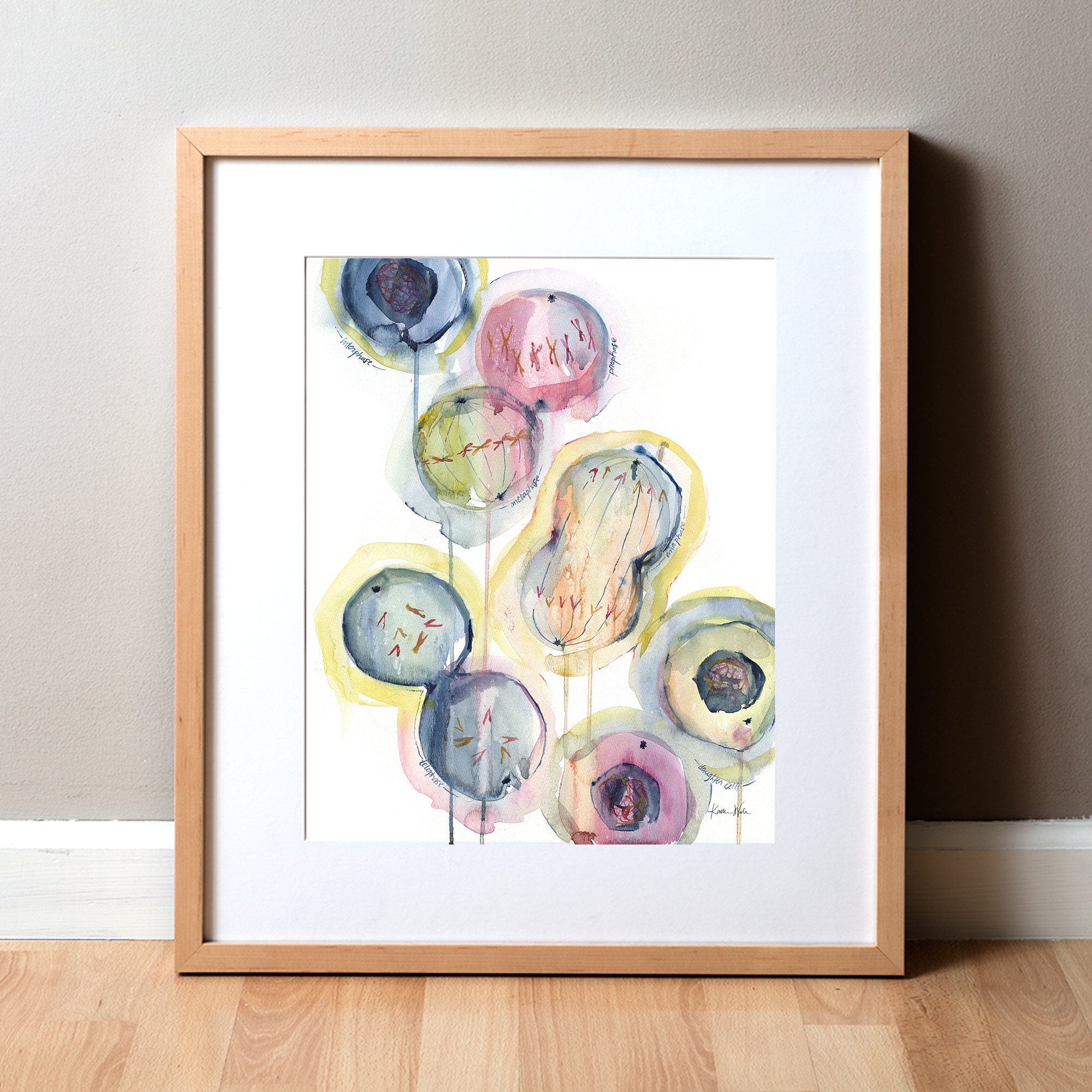The image presents a framed watercolor painting depicting a collection of colorful balloons with thin strings. The balloons are in various hues, including shades of pink, purple, yellow, light blue, and a touch of green. Notably, some balloons feature inner circles reminiscent of Tootsie Pop candy, and one balloon exhibits a peanut-like shape, diverging from the typically round forms. The scene is accentuated by a light-colored wood frame, bordered by a white cardboard matting. This framed artwork is positioned against a light gray plaster wall, with a white baseboard and light-colored finished wooden flooring completing the setting.